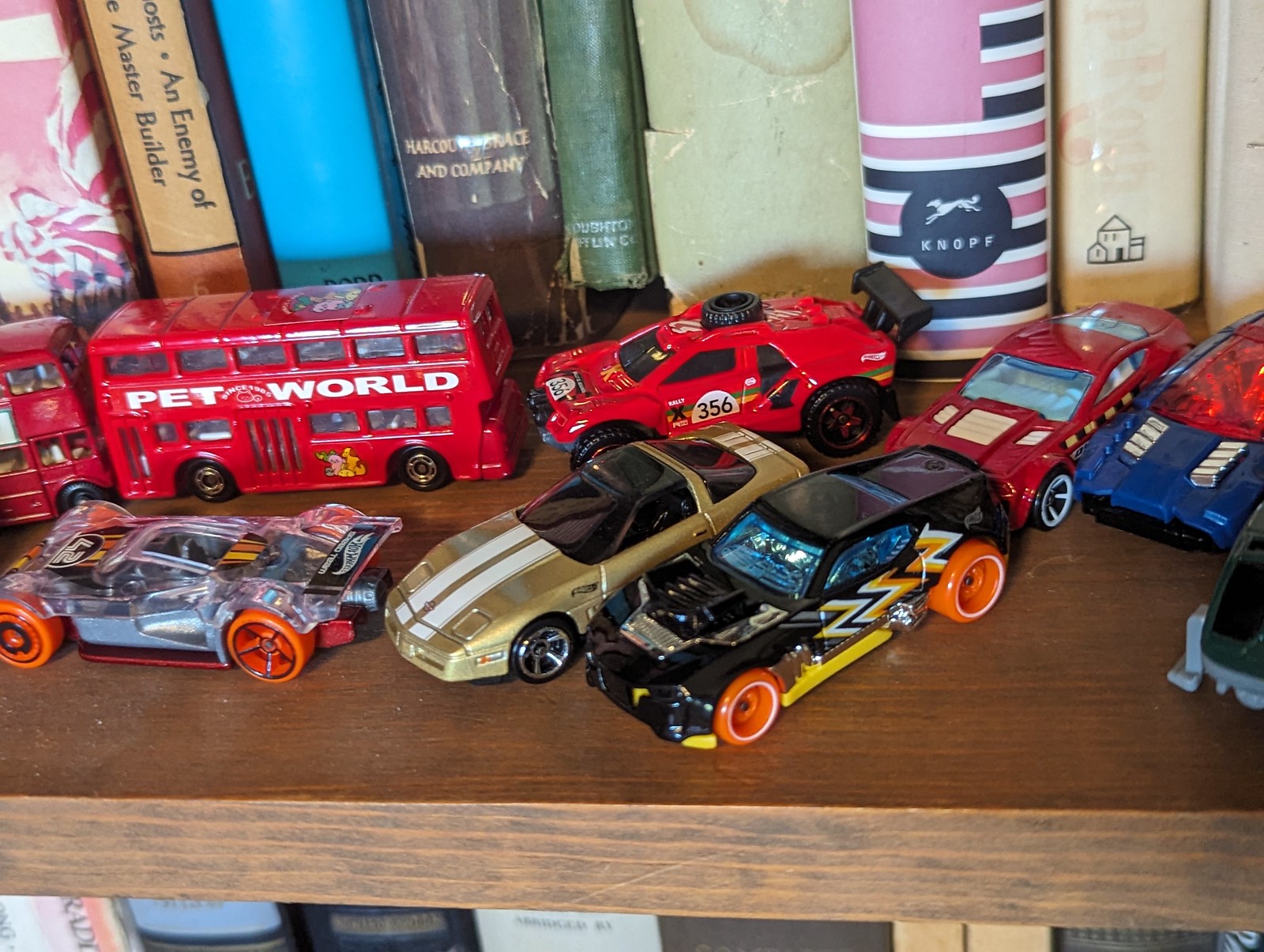This photograph features a nearly perfectly square wooden bookshelf. The bookshelf showcases a diverse collection of books arranged neatly along two visible shelves, with a vibrant assortment of spines in colors such as pink, blue, brown, tan, cream, and green. Titles such as "An Enemy of Master Builder," "Hardcore Grace and Company," and "KNOPF" are discernible among the books, while others have indistinguishable or blank bindings.

The central focal point of the image is the display of toy cars and buses adorning the shelf. Notably, there are two red double-decker buses labeled "Pet World," adorned with pet images. The toy cars include a variety of designs: a red sports car with a black spoiler and black wheels, another red car with white detailing on the hood, a blue car with a red top, a black sports car featuring orange wheels and yellow and orange accents, a gold car with white racing stripes, and a distinctive clear car with black, orange, and red markings, completed with orange wheels. 

Below this shelf, additional books can be seen, hinting at the extended literary collection housed in this piece of furniture. The overall arrangement offers a charming interplay between literary and playful elements, creating a visually captivating and detailed scene.